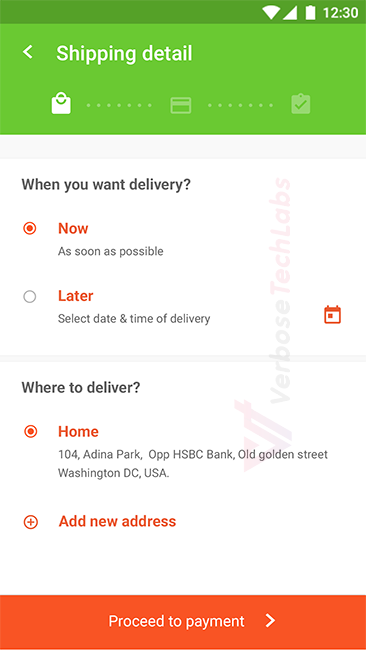**Caption:**
Screenshot of a Shopping App's Shipping Details Page

Description:
This screenshot, likely taken on an Android smartphone as suggested by the status bar icons, captures the "Shipping Details" section of a shopping app by Verbose Tech Labs. The status bar at the top shows the current time as 12:30 PM, with full battery, strong Wi-Fi, and network signals. Below the green header labeled "Shipping Detail," users are prompted to choose their delivery preference between "Now" (as soon as possible) and "Later," the latter offering a clickable calendar for selecting a specific date and time.

Under the delivery options, the user can specify the delivery location. The default address listed is "104, ADINA Park, OPP HSBC Bank, Old Golden Street, Washington DC, USA," with an option to add a new address.

At the bottom of the screen, an orange button labeled "Proceed to Payment" spans the width of the display, inviting users to finalize their purchase.

The screenshot was captured in standard (not dark) mode, with a watermark at the bottom featuring the logo of Verbose Tech Labs, which includes an interlinked "V" and "T."

(Note: The specific app platform cannot be identified from the screenshot.)